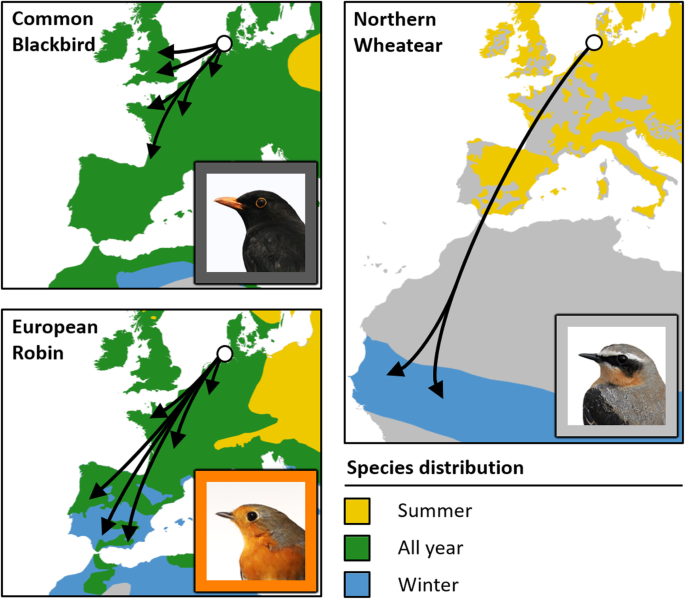The image presents an animated chart detailing the species distribution and migration patterns of three types of birds: the Common Blackbird, the Northern Wheatear, and the European Robin. The chart is divided into three main squares, each dedicated to one bird species. In the upper left corner, the Common Blackbird's square features green shapes denoting its year-round habitat and a white circle with black arrows indicating its migratory directions. The bird is illustrated in side profile with a black coat and an orange beak. To its right, the Northern Wheatear's square incorporates swatches of yellow, gray, and light blue to depict various landmasses, alongside another white circle with a black line branching into two arrows, illustrating its migration routes. This bird is depicted with a light gray, black, and white coloration. In the bottom left square, the European Robin is shown with green, yellow, and light blue sections representing different seasons and a white circle with black arrows marking its migration. The European Robin is illustrated with a light gold face, gray body, and dark eyes. In the bottom right corner of the image, black text reads "species distribution," followed by a color key: yellow for summer, green for all year, and light blue for winter. The chart effectively uses color-coded regions and directional arrows to convey the birds' seasonal movements.